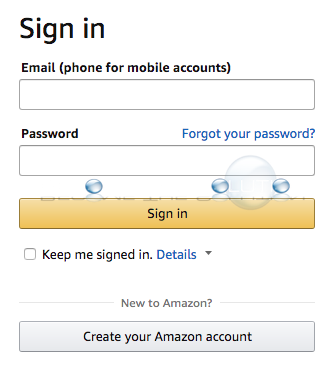The image depicts the Amazon login page, characterized by its minimalistic and predominantly textual design against a white background. At the top, in bold black text, it reads "Sign In." Below that, a line of text prompts users to enter their "Email (phone for mobile accounts)", followed by an empty input box for users to type in their information. 

Next, "Password" is written in black text, with "Forgot your password?" positioned horizontally to the right, in blue, indicating a clickable link for password assistance. Below these elements, there is another empty input box for entering the password.

Following the password field, there is a notable yellow-gold button labeled "Sign In" in black text, signaling it is clickable. Beneath this, there is an unchecked checkbox labeled “Keep me signed in.” To the right of this checkbox, the word “Details” appears in blue, suggesting it is a clickable link, accompanied by a down arrow, also likely clickable.

Further down, a question in black text reads “New to Amazon?” Underneath, another clickable box is presented with the text “Create your Amazon account” in black.